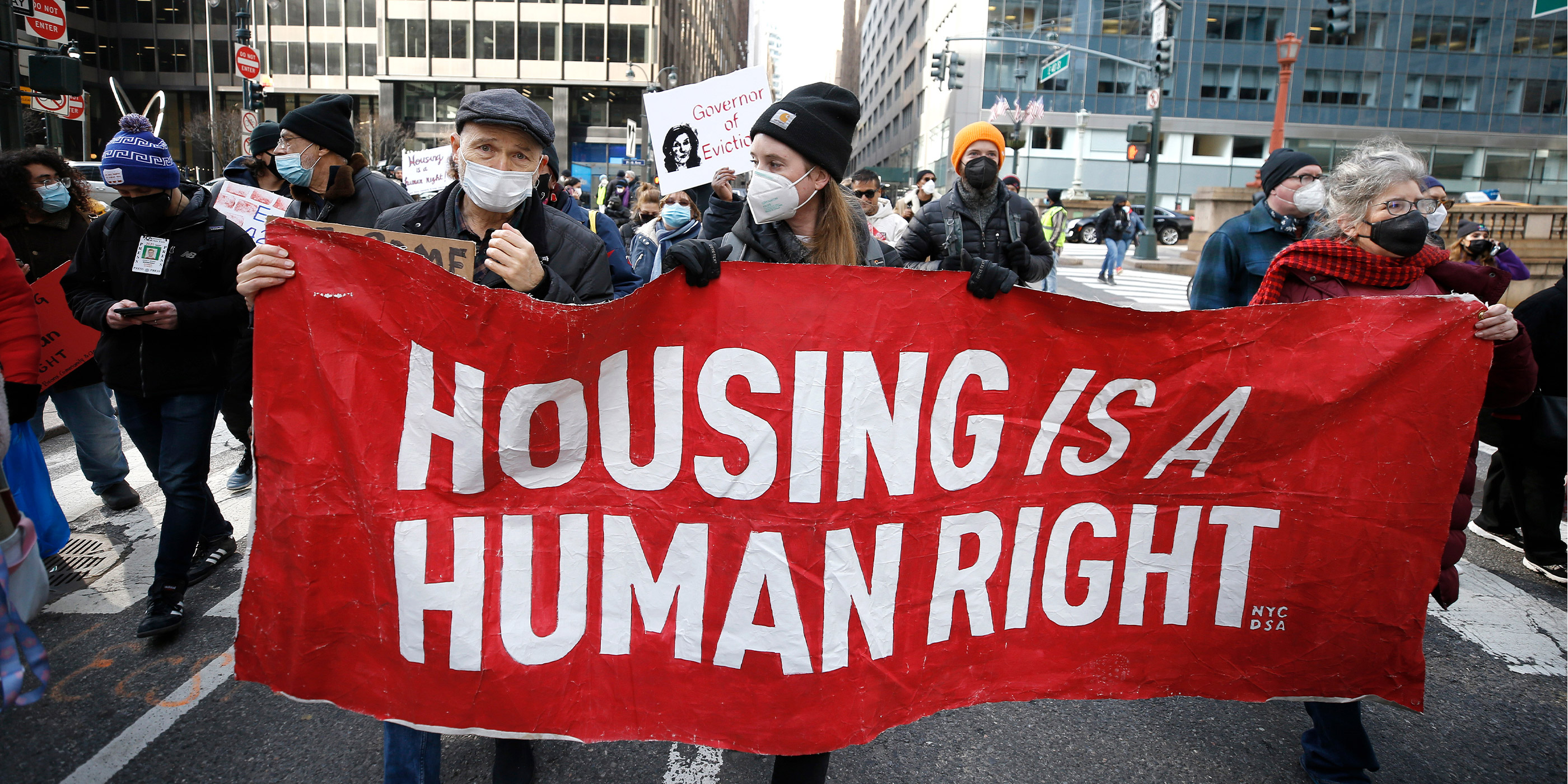This photograph captures a protest march on a city street, likely in New York City. At the forefront, three individuals are prominently holding a large red banner with bold white text that reads "Housing is a Human Right" along with smaller text "NYC" next to the 'T' in "Right." The trio includes an older woman with gray hair on the right, an older gray-haired man on the left, and a person with long hair and a black beanie in the center. They are crossing an intersection, with a street sign in the distance indicating East 42nd Street. Surrounding them are additional protesters, many of whom are wearing masks, indicative of a COVID-19 era protest. Some other signs are visible, one notably with the message "Governor of Eviction" and a black-and-white photo of a woman. The scene is framed by tall city buildings, street posts, traffic lights, and street lamps, enhancing the urban atmosphere. The participants are dressed in cold weather attire, suggesting the protest took place during a colder season.